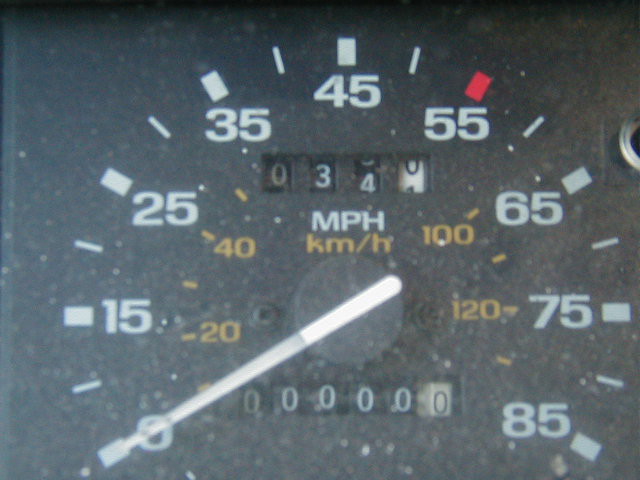The image showcases an analog speedometer dial within a car, exhibiting a prominently used and aged appearance. Speckles of dust, dirt, and debris are visible on the surface of the gauge and the glass covering it, indicating a lack of recent cleaning. The plastic casing surrounding the dial is heavily coated with dust, further contributing to its worn-out look.

The speedometer displays dual measurement units: the main outer dial reading up to 85 miles per hour (mph), while the inner indicators reach up to 120 kilometers per hour (km/h). The odometer, reset to zero, underscores that the gauge has been reset at some point, hinting at its pre-owned condition. Above the odometer, the trip mileage shows a figure of 34.5 miles, recorded between the zero and one mark.

A stark white pointer stands out against the dark gray background of the dial, adding to the clarity of the well-worn instrument despite the grime. The lens covering the speedometer is notably soiled and dirty, emphasizing the gauge's extensive use and the accumulation of particulate matter over time.